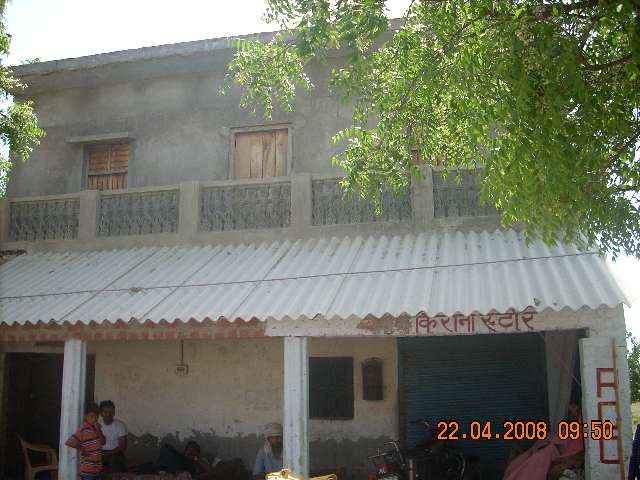This is a photograph of a dilapidated two-story white house, with a metal tin roof showing signs of wear. The second floor features two windows and a balcony, while the first floor has an awning extending over a porch area. There is graffiti or spray-painted writing underneath the awning. In front of the house, there are several individuals: two men on the far left, two in the middle, and possibly another man on the far right. Additionally, two people can be seen standing under the roof, leaning against a beam. A large tree is positioned in front of the house, and the photograph was taken on April 22, 2008, at 9:50 a.m., set against a white sky. Peeling paint further adds to the ramshackle appearance of the structure.